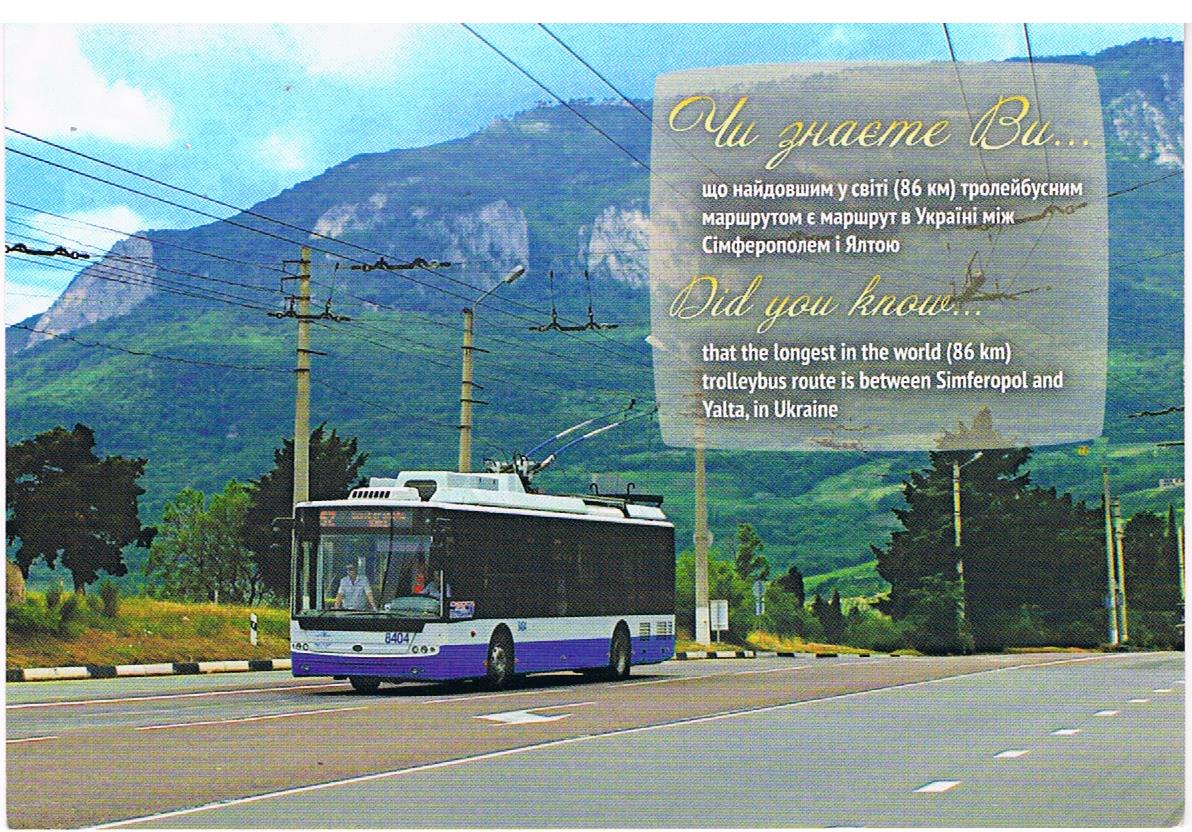This grainy photograph captures an electric-powered tourist bus traveling on a road, set against the backdrop of a tall, grassy mountain that resembles tropical foliage common to locations like Hawaii, although it is actually in Ukraine. The bus, distinct with its black area around the windows, white top, and blue striped bottom, appears to be older and features two arm bars connecting to overhead trolley wires. The central figure of the image, the bus is heading towards the right, presenting a slight diagonal angle where two occupants are visible through the front windshield—one standing and one seated behind the steering wheel. The surrounding scenery is rich with greenery, including trees, shrubs, and expansive grassy areas, accentuated by blue sky and white clouds. The photograph includes an informative text box in Cyrillic and English, noting, "Did you know that the longest in the world 86 kilometer trolley bus route is between Simferopol and Yalta in Ukraine?" This detail confirms the location and historical context of the image, enhancing the vintage feel indicated by its graininess and dated aesthetic. The road depicted is a multi-lane country road with visible power lines, positioned centrally in the composition, which guides the viewer's eye across the serene yet intriguing landscape.